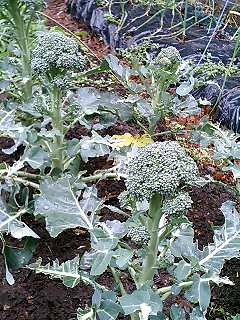This photograph captures a small, vertically-oriented garden plot viewed from above. Central to the image are several broccoli plants, identifiable by their big cabbage-like leaves and light, chalky green stalks. Among them, three broccoli heads are visible, though they appear unhealthy and ravaged by pests, with bite marks on the leaves. The leafy greens exhibit a silvery-green hue with occasional splashes of brown mulch and dirt. In the background, interspersed among the broccoli, are plants with purple leaves, possibly kale or other greens. The scene suggests a densely packed garden where various vegetables overlap each other, highlighted against a moderately rich, brown soil. The photograph's angle is steeply tilted to the right, creating a dynamic view that emphasizes the garden's texture and color variations. Hints of red clay and scattered dead materials are visible in the background, contributing to the organic, somewhat unkempt appearance of this community garden plot.